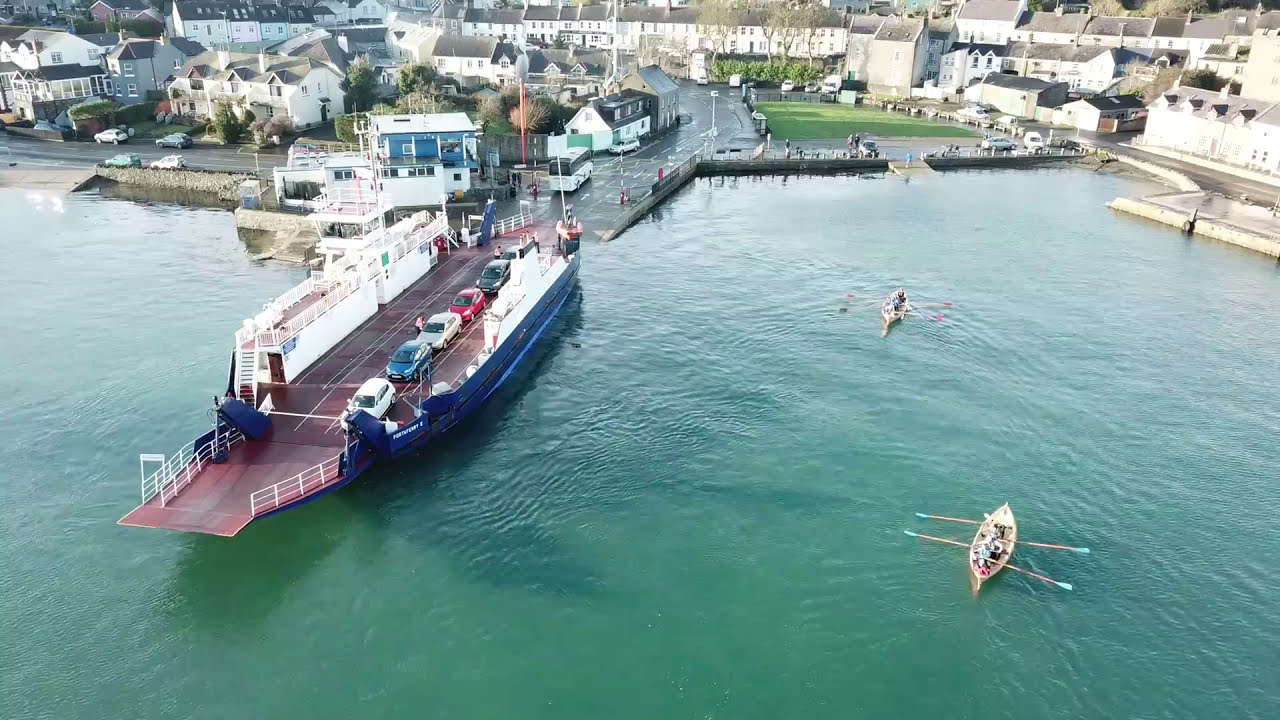In the image, we see a greenish-blue body of water that appears to be a river or canal, harboring various watercraft and overlooked by an array of houses. Two canoes, each with two individuals, one paddling from the front and the other from the back, navigate the water. The canoe in the bottom right is distinct with teal-colored fins. To the left side of the image, a large ferry or barge, painted dark blue near the waterline, is laden with cars, including a white, blue, silver, red, green, and gray one, and lined with a white barrier against its amber-colored deck. This ferry is positioned near a typical gray asphalt road, allowing vehicles to drive directly onto it. In the background, an orderly collection of mostly two-story houses with white walls and gray roofs rise behind this busy waterfront scene. The ferry dock is also noted to have a smaller area for people to board, and a bus is parked nearby, adding to the bustling atmosphere.